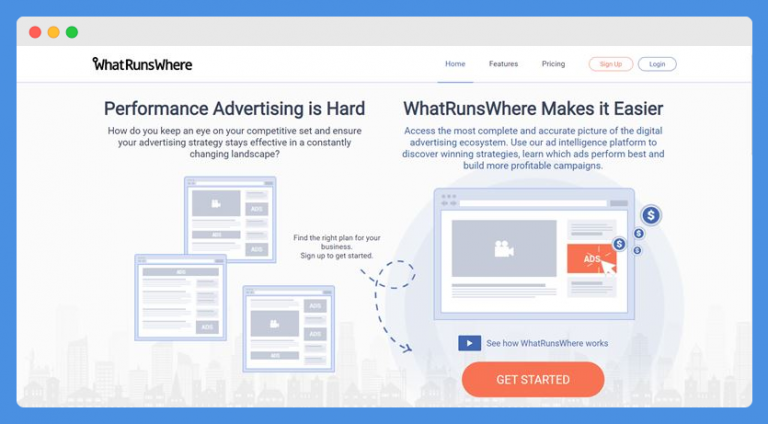The image showcases the homepage of the "What Runs Where" website, which appears to be a platform dedicated to optimizing advertising strategies for private websites. The interface is cleanly organized with a blue navigation bar at the top.

On the left side of this blue bar, there are three colorful buttons in red, yellow, and green. Directly beneath these buttons, a stylized logo featuring the name "What Runs Where" is prominently displayed in a cursive font. To the right of the logo, the navigation menu includes links labeled Home, Features, Pricing, Sign Up, and Log In.

Below the navigation elements, a bold headline reads "Performance Advertising is Hard." This is followed by an insightful question: "How do you keep an eye on your competitive set and ensure your advertising strategy stays effective in a constantly changing landscape?" To address these questions, the layout contains three distinct informational boxes with corresponding content. An arrow on the right side beckons the user to proceed further.

The following section, titled "What Runs Where makes it easier," explains the benefits of using their ad intelligence platform. It describes the service as providing the most comprehensive and accurate view of the digital advertising ecosystem, enabling users to discover successful strategies, identify high-performing ads, and develop more profitable campaigns.

Directly beneath this explanation is a visual representation of a website within a box. Further down, a prompt reads "See how What Runs Where works," leading to an inviting orange button labeled "Get Started" in vibrant yellow lettering.